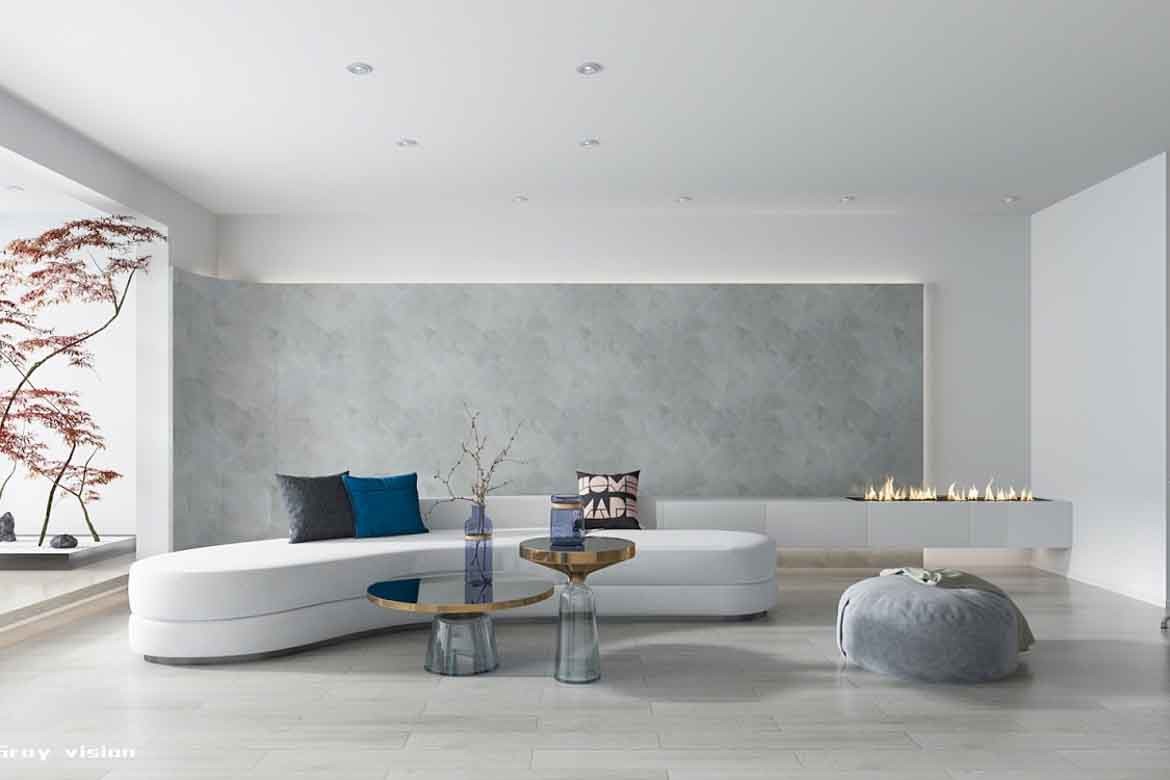Capture the sophisticated minimalism of this ultra-modern living room, a color photograph in landscape orientation that epitomizes contemporary design. The walls are pristine white, complemented by a light gray textural backdrop two-thirds up the rear wall. At the center stands a kidney-shaped sofa adorned with a single small backrest and no arms, accessorized with black and blue throw pillows. Complementing the sofa are two distinctive mushroom-shaped coffee tables with clear bottoms and brass-banded round tops.

To the rear right, there's a sleek gas fireplace beneath the gray backdrop, flanked by a large, inviting round gray ottoman. The light gray wood tone plank flooring lends a warm yet minimalist touch to the space. On the far-left side, a case opening reveals a glimpse of a Japanese red maple tree, enhancing the room's serene atmosphere with an element of natural beauty.

A subtle, textural theme permeates the space through details like the word "vision" in the bottom left-hand corner of the photo, possibly alluding to the brand or the image's curated essence. Floating islands of seating options, including a stylishly understated beanbag chair on the right side, provide varied lounging possibilities. Overhead, recessed lighting ensures a clean, well-lit environment, accentuating the room's elements, from the bonsai decor tree in an adjoining room to the minimalist yet inviting lounging spaces.